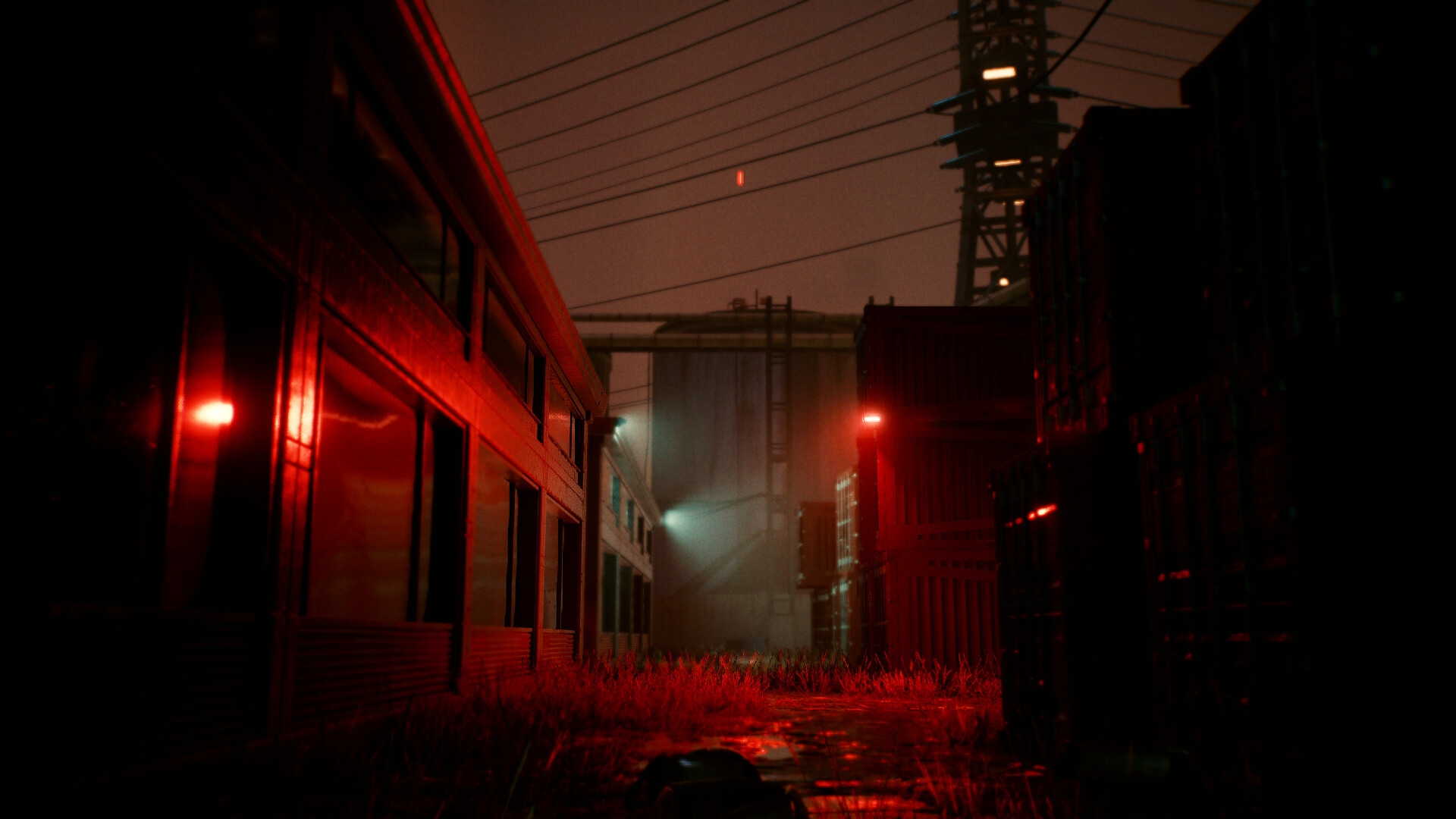The image depicts an industrial section of a city at nighttime, enveloped in a dark, maroon-colored sky. The scene is primarily lit by a bright red light emanating from the corner of stacked shipping containers on the right side of the image. These large shipping containers cast dark shadows both on the right and left sides of the photograph.

To the left, a warehouse with numerous closed loading bay doors is heavily bathed in the red glow from the light near the containers. This red illumination also spreads across the ground below. In the center background of the photograph, a large gray silo rises, casting a gloomy presence. Farther to the right, towering above, is an electrical transformer interwoven with numerous power lines.

The backdrop reveals additional buildings, one to the left with large, opaque windows, suggesting a two-story structure. In contrast, the building to the right remains shrouded in darkness, devoid of visible details. In the foreground, the ground shows patches of grass struggling to grow amidst the industrial setting. The entire scene is framed under the night sky, which holds a faint glimmer of light, contributing to the hauntingly industrial yet eerily illuminated ambiance.